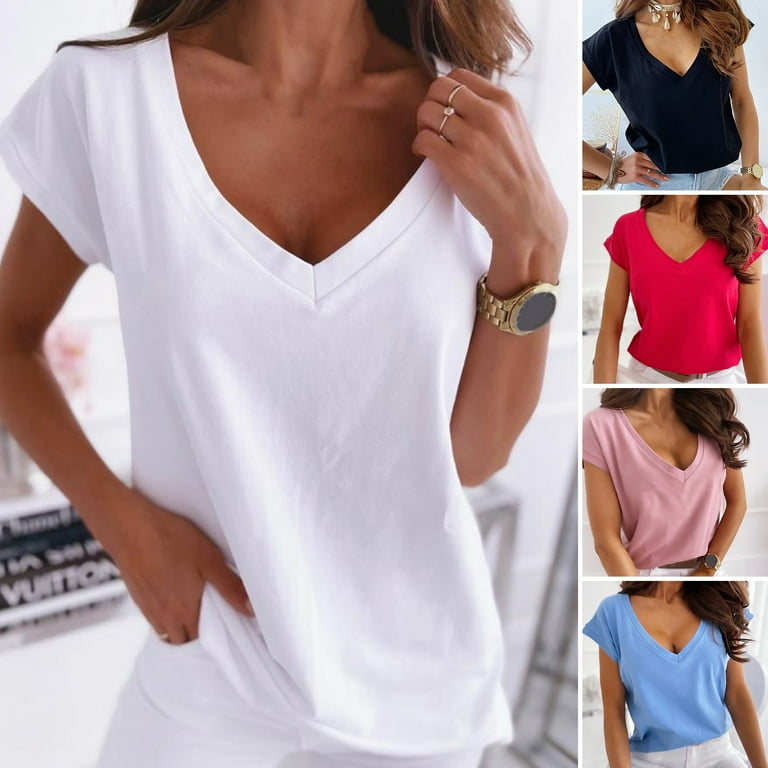This is a detailed promotional image showcasing a woman modeling a v-neck t-shirt in various colors. The main photograph on the left highlights a tan, skinny woman with shoulder-length brown hair, cropped from the neck down to the waist. She is wearing a loose-fitting, low-cut white v-neck shirt paired with white pants. Her left arm, adorned with a gold wristwatch and two gold rings, is raised to her left shoulder, while her right hand rests in her pant pocket. 

To the right of the main photo, there is a vertical strip containing four smaller images of the same woman, each modeling the same shirt in different colors. In the top right image, she poses in a black v-neck shirt with a hand on her hip. The second image down features her in a reddish-pink v-neck with her hands down to her sides. The third image shows the shirt in a pale pink hue, and in the fourth and final image, she models a light blue v-neck, accentuating the shirt's low-cut design with noticeable cleavage.